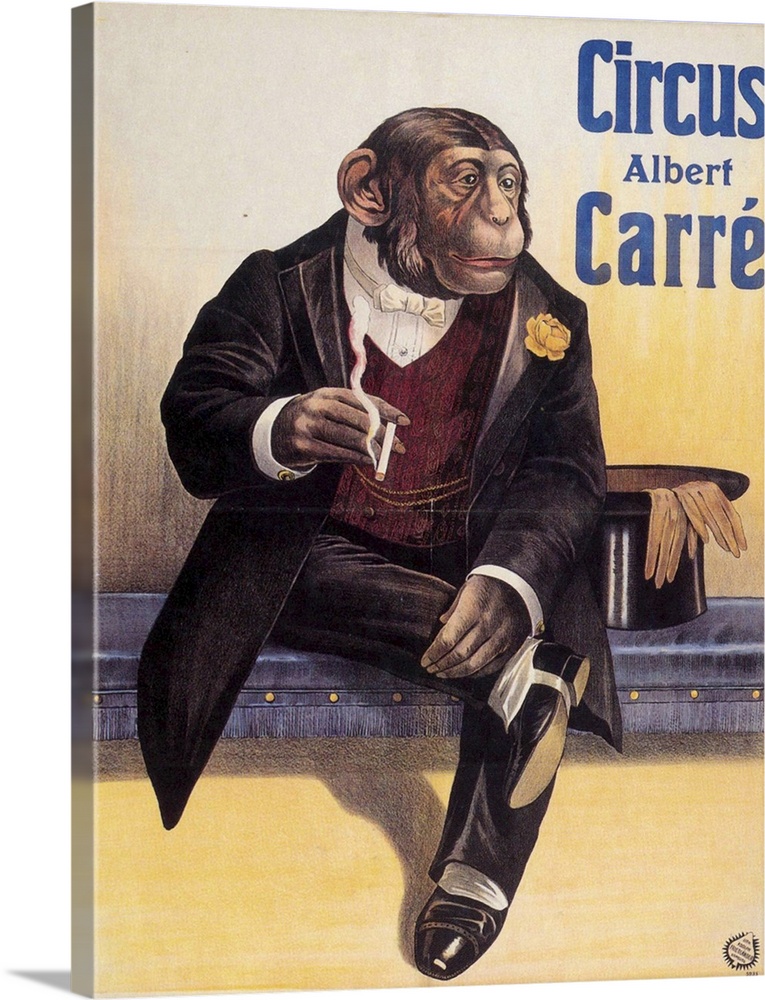This detailed illustration depicts a chimpanzee in a sophisticated attire, comfortably seated on a navy blue upholstered bench. The chimpanzee, with neatly combed dark brown hair, light brown face, ears, and hands, exudes an air of refinement. He is dressed impeccably in a black tuxedo jacket adorned with a yellow corsage on the left lapel, a red vest with a pocket chain, a white dress shirt beneath, and a white bow tie. His black pants are accented by black shoes with white spats.

The chimpanzee's right leg is casually crossed over his left knee, with his left hand resting on his ankle and his right hand holding a cigarette, which he is smoking. To his right, on the bench, lies a black top hat turned upside down with two white leather gloves draped over its brim.

The background features a gradient from gray to yellow on the floor beneath the bench. Text in blue at the upper right-hand corner reads "Circus Albert Carré," suggesting that this is possibly an advertisement for a circus. The overall composition evokes a sense of whimsical elegance, with the chimpanzee appearing relaxed yet dignified in his setting.